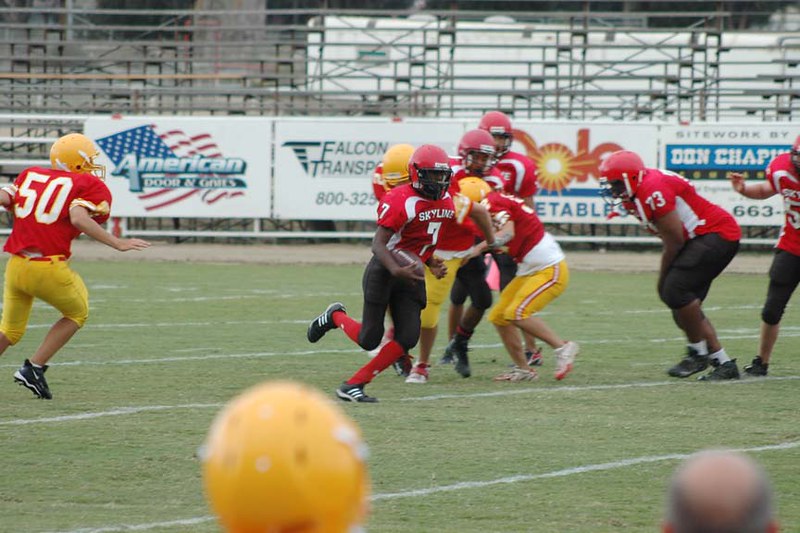A dynamic moment captured from a junior or middle school football match features a running back, prominently centered, wearing the number 7 jersey. He is seen charging down the field with determination. The two opposing teams are easily distinguishable: one team dons yellow helmets and yellow pants, while their rivals sport red helmets paired with black pants. In the backdrop, the stands are visible, lined with enthusiastic spectators and colorful banners promoting local businesses such as American Door and Grills, Falcon Transports, and several others, adding to the lively atmosphere of the match.